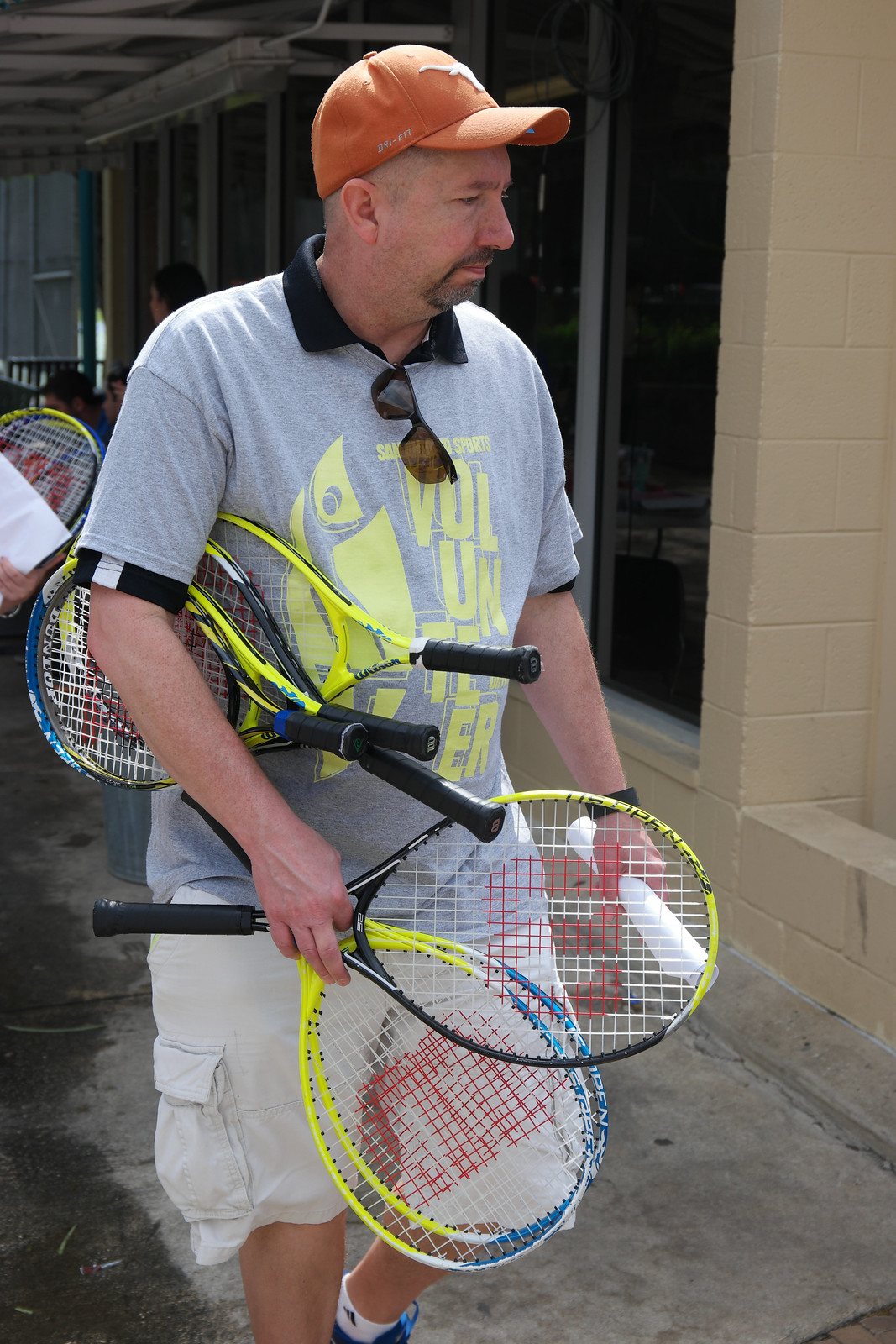In this image, we see a tall, middle-aged white man with a goatee, walking down an outdoor hallway with brick walls and large plate glass windows, all set against a concrete floor. He is wearing a gray t-shirt over a black polo shirt, with an orange Texas Longhorn baseball cap on his head. His khaki cargo shorts complement the casual outfit, and he has a black watch on his left wrist. The man is holding approximately six tennis rackets—three under his arm and three in one hand. These yellow Wilson rackets, marked with a red "W" and featuring black handles, suggest his involvement with the sport. Additionally, he is carrying a white rolled-up piece of paper and has a pair of sunglasses hanging from his shirt, indicating a preoccupied demeanor as he looks downward. Behind him, a person is also seen holding a racket, adding to the scene's athletic theme.